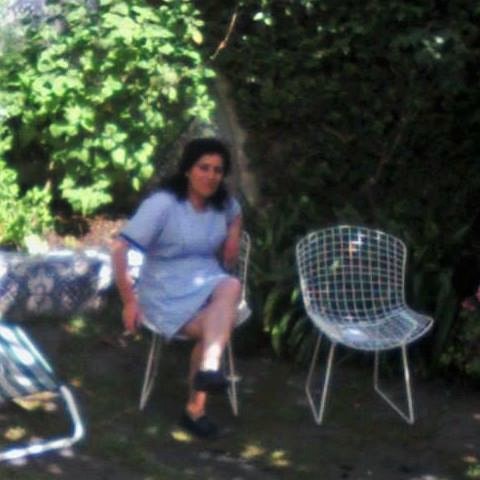In this outdoor scene, a light-skinned woman with short black hair is sitting in a white metal lawn chair that features multicolored squares in shades of dark blue, dark green, red, and orange. She wears a short-sleeved, light blue dress with dark blue accents on the sleeves and waist, paired with black shoes. Next to her is an identical white chair, and a folded beach chair lies on the ground to her left. A small footstool with dark blue, green, and white stripes supported by white painted steel is also on her left but is partly obscured by shade. The woman appears to be holding a cigarette in her right hand. The background showcases a mix of light green and dark green foliage, with sunlight casting a glow in the top left corner. The ground beneath her seems to be a dirt area with scattered short green grass. A partially visible box with blue, green, and white splotches is also present in the scene, contributing to the vibrant yet calm outdoor atmosphere.